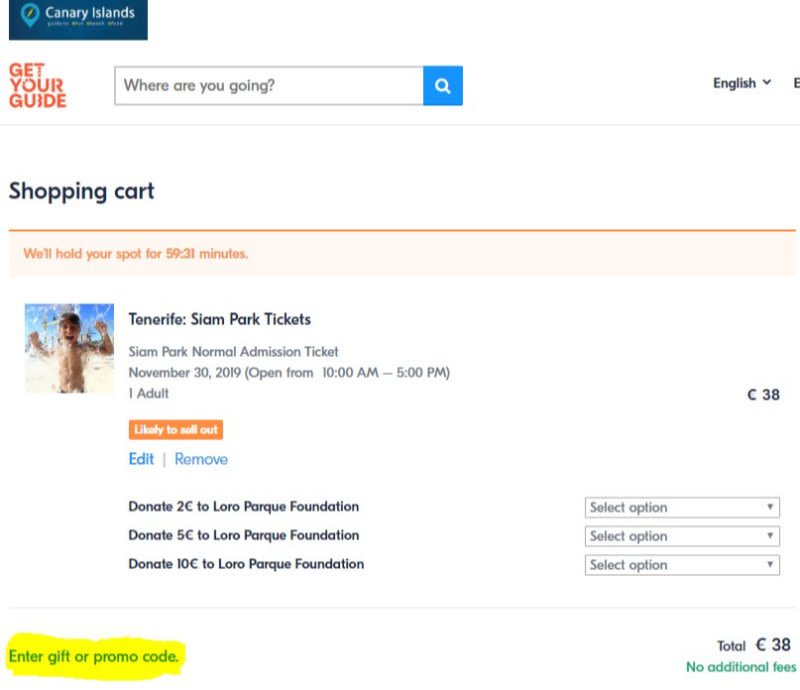The image depicts a website interface for booking activities in the Canary Islands. In the top left corner, a blue panel displays an icon alongside the text "Canary Islands." Beneath this, on the left-hand side, large capital letters in orange spell out "Get Your Guide," accompanied by a search box where users can input their desired destination. On the right-hand side of the top panel, there's an option to select the site’s display language.

Underneath, on the left-hand side, a title reads "Shopping Cart." An orange banner below it indicates that the website will hold your spot for 59:31 minutes. The shopping cart contains a picture of a child and details about "Tenerife Siam Park tickets," priced at 38 euros for one adult for the date November 30, 2019. An orange panel beneath this information notes that the tickets are likely to sell out. Additional blue buttons labeled "edit" and "remove" allow for modifications to the booking. 

A dropdown menu offers the option to make donations of 2, 5, or 10 euros to the Laurel Park Foundation. The total price, without any additional fees, is currently 38 euros. At the bottom left corner, there's a section labeled "enter gift or promo code," highlighted with a bright yellow marker to draw attention.